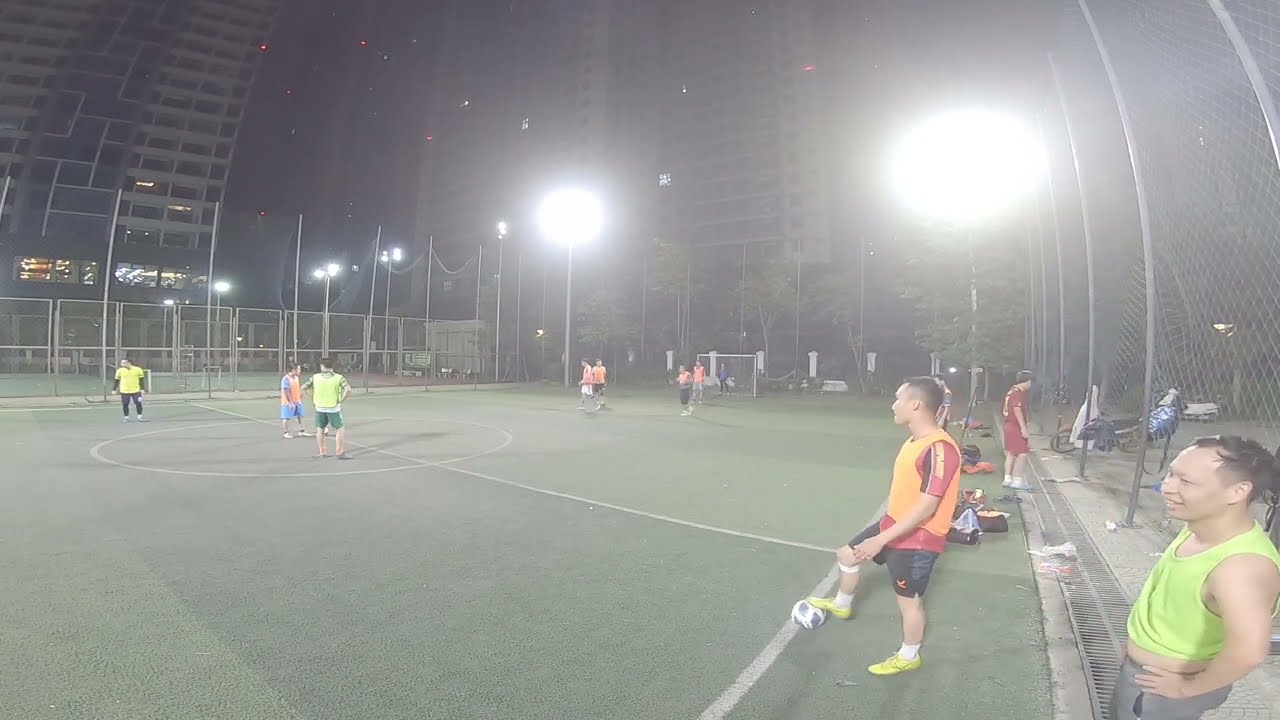In this image, we see an outdoor soccer game being played at night, set in the midst of a bustling cityscape. The soccer field, likely made of artificial turf, is brightly lit and surrounded by tall apartment buildings that rise up to about 12 floors, emphasizing the urban environment. At the bottom of the image, the center of the field is depicted, with a goal visible off-center and a cage or gate on both sides to keep the ball contained. Several players are gathered around, with three individuals at the midfield circle preparing for the game. One player at the right side of the image has their foot on a soccer ball, poised for action. The players appear to be wearing plain intramural-style jerseys; some in orange tank tops over red shirts, while others don neon yellow vests. The athletes, who seem to be of Asian descent, are dressed in t-shirts, shorts, and sneakers, with one player wearing only the jersey without an undershirt. The game exudes a vibrant, communal atmosphere under the overhead lights, devoid of any text or signage, and features a rich palette of colors including green, yellow, orange, red, black, tan, lime green, white, and gray.